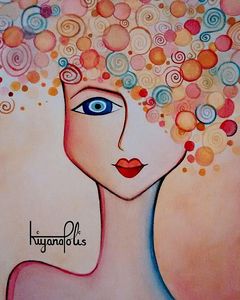The image is an abstract painting of a woman’s face, distinguished by its vibrant and colorful details. The composition begins around the shoulder level, showing the neck and head of the woman. The right side of the neck is outlined in blue, while the left side in red. The face features highly feminine characteristics, including bright red lips and a distinctive nose. The painting depicts only one eye, located on the left side, which is detailed with concentric circles – a blue iris with a white circle, a darker blue outline, and a black pupil.

The woman’s hair is illustrated through an intricate array of spiral and swirl patterns, representing her hair in a dynamic and colorful fashion. These spirals and swirls are a medley of blue, red, pink, orange, yellow, and shades of white. The overall face shape appears to be heart or diamond-shaped, accentuating her delicate features. The image includes text that reads "KINOPOLIS," albeit not in legible English.

The vibrant color palette includes shades of blue, red, pink, orange, yellow, and various shades of white and blue, lending the image a vivid and dynamic feel. The playful and colorful swirls create a visually captivating representation of the woman's hair, enhancing the abstract and artistic nature of the painting.